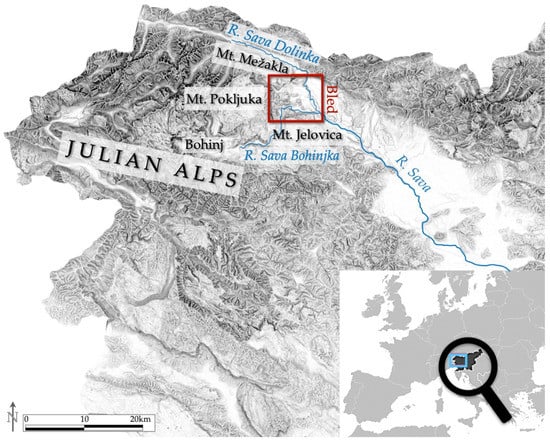This black and white map highlights the Julian Alps, characterized by detailed terrain features and variations in shading to depict relief. At its center, a specific region outlined in red is labeled "Bled," signifying an area of interest. Prominent geographical markers include the Sava-Bohinjka River, Sava-Dolinka River, Mount Jelovica, Mount Mežakla, and Mount Pokljuka, along with Bohinj, although Bohinj is not identified as a mountain. A legend in the lower right corner features a magnifying glass zooming in on this specific area, pinpointing its larger European context with nearby Italy. Additionally, the map's lower section presents a scale of 0-20 km and a compass rose indicating north, lending to its navigational utility. The map appears either hand-drawn or designed with an old-fashioned aesthetic, enhancing its detailed and historic look.